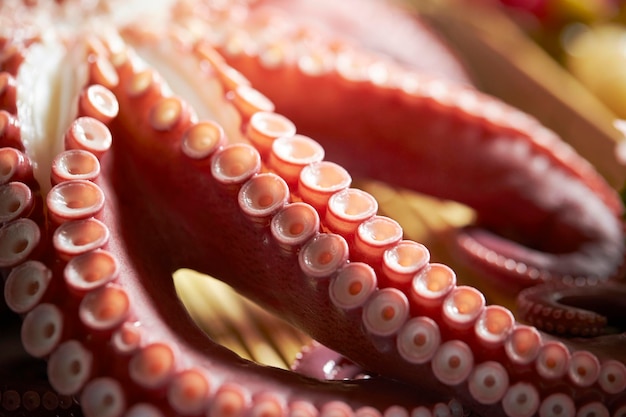This close-up photograph captures the intricate details of an octopus's pink tentacles. The focus is on three tentacles coiling towards the bottom right of the image, each lined with hundreds of tiny, lighter pink suckers that resemble small white circles with little holes in the center. The tentacles, resembling finger-like expansions, are slightly curled at the tips and extend gracefully. In the top right corner, the octopus's belly is visible, showcasing more of its pink hue. The octopus is resting on an out-of-focus surface, identified as a type of bamboo tray, enhancing the clarity and texture of the tentacles and their array of suckers.